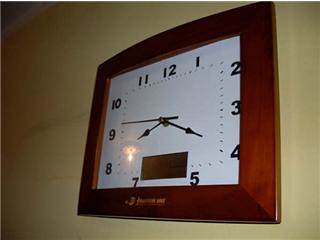The image depicts a unique square clock hanging on a yellowish-white wall in a relatively dimly lit room. The clock features a wooden border and a white face with black numbers for each hour position, except for where the 6 would be, which is replaced by a small digital display. The time shown is approximately 8:20, as indicated by the three slender hands—hour, minute, and second—each with spade-shaped tips. A small nameplate or placard is also visible on the front of the clock, adding to its distinct design.